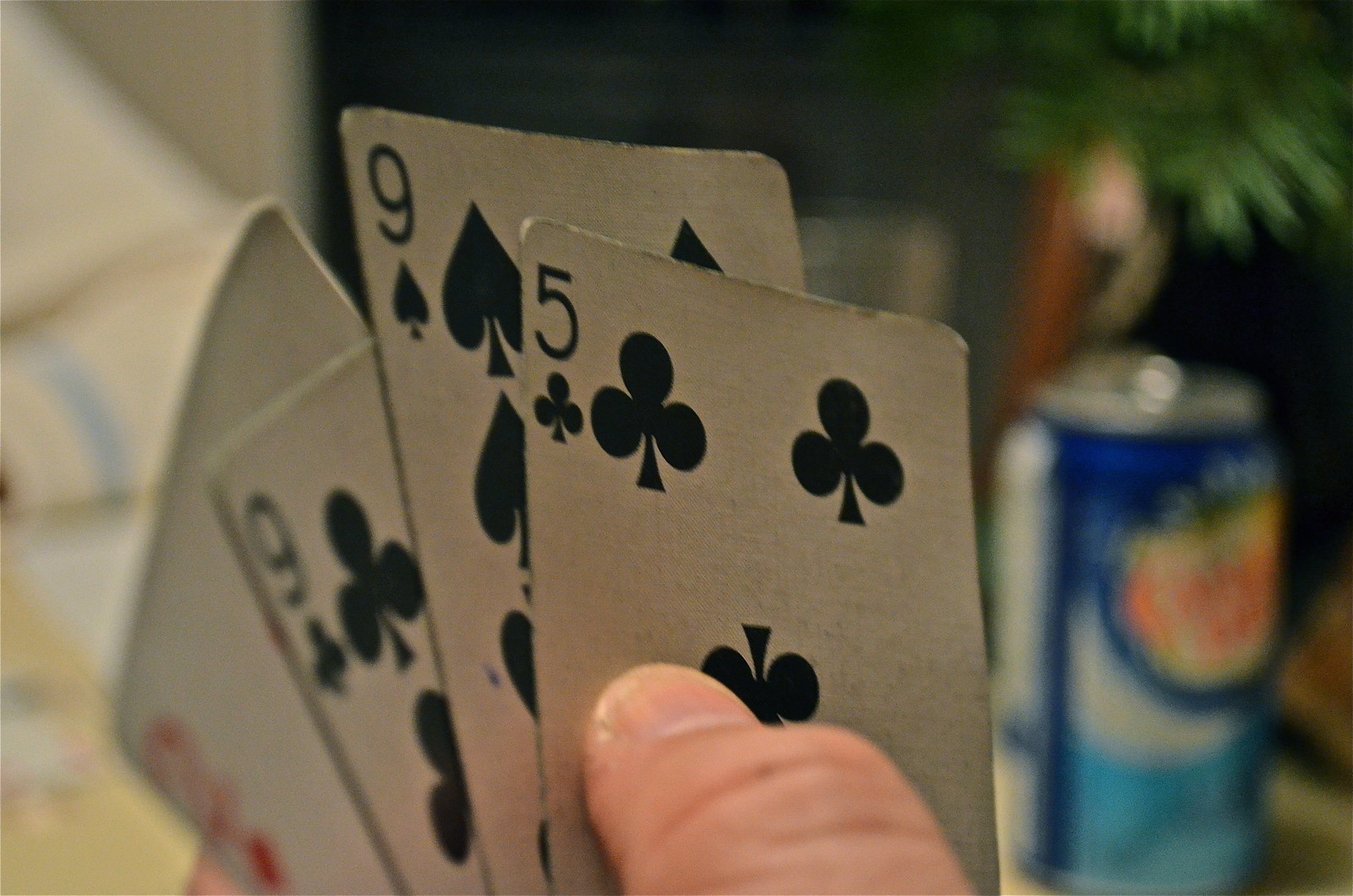A person is holding a fan of playing cards prominently in the foreground, capturing the thumb in sharp focus while the background remains blurred. The hand displays a sequence of cards angled from left to right: the Five of Clubs, the Nine of Spades, the Nine of Clubs, another Nine of Spades, and the Two of Diamonds, which progressively become out of focus. Only the person's thumb is visible, bent slightly, with a short, trimmed nail and a small hangnail visible on the side. There is also a white mark, possibly a healing scab, in the crease of the thumb. The background features a dark blue, light blue, and white can with a tree design on it to the right, and a table against a white wall partially visible on the left. The overall scene is set against a blurred backdrop, keeping the viewer's attention on the hand of cards.